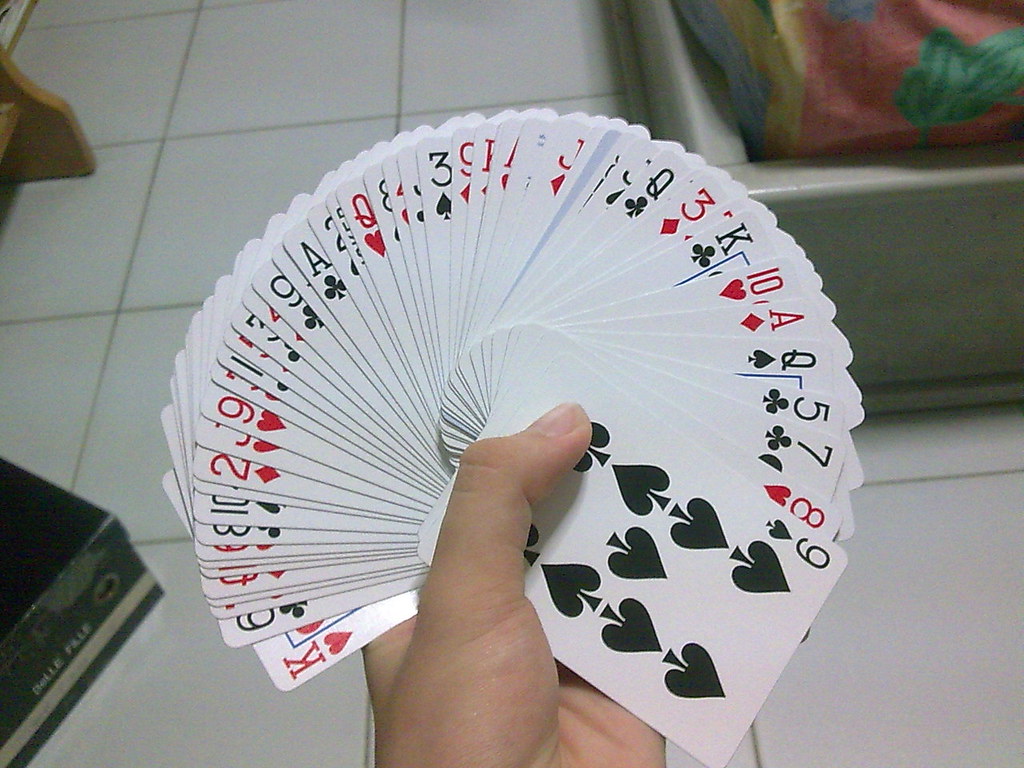In a modest bedroom setting, a man's hands take center stage as he demonstrates a card trick. He holds a deck of playing cards, expertly fanning them out with his thumb. The top card is an ace of nines, prominently displayed. The cards, a blend of red and black suits, contrast against the white tile floor visible behind his hands. On the floor rests a bed with colorful sheets in shades of pink, yellow, and green. To the left, a shoe box and a piece of wooden furniture add to the room's simple decor. The photograph captures an unembellished moment, focusing on the intricacies of the card trick amidst the everyday surroundings.